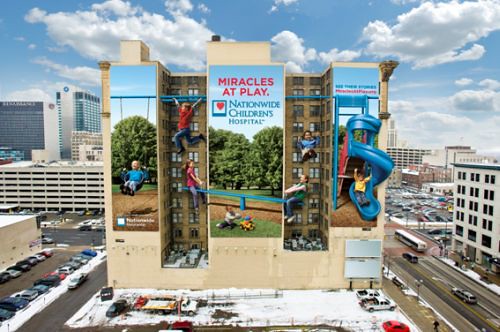The image depicts an aerial view of a large metropolitan area featuring a prominent building adorned with an extensive mural. This structure, identified as Nationwide Children's Hospital, boasts a tan exterior with intricate architectural features, including sections that jut in and out. The mural, titled "Miracles at Play," spans the building's exterior and showcases children engaging in various playground activities. On the left side, a child is on a swing set, while to the right, another child slides down a blue, curvy slide, clad in a yellow shirt. The mural also includes depictions of children playing on monkey bars, a teeter-totter, and other playground equipment. Surrounding the hospital are busy city streets with cars and additional buildings, emphasizing its downtown location. Below the hospital, parking lots scattered with snow are visible, contributing to the urban landscape. Above, the sky is partly cloudy, with patches of blue and fluffy white and gray clouds. This detailed and vibrant scene captures the essence of a bustling city center with a focus on children's healthcare and play.